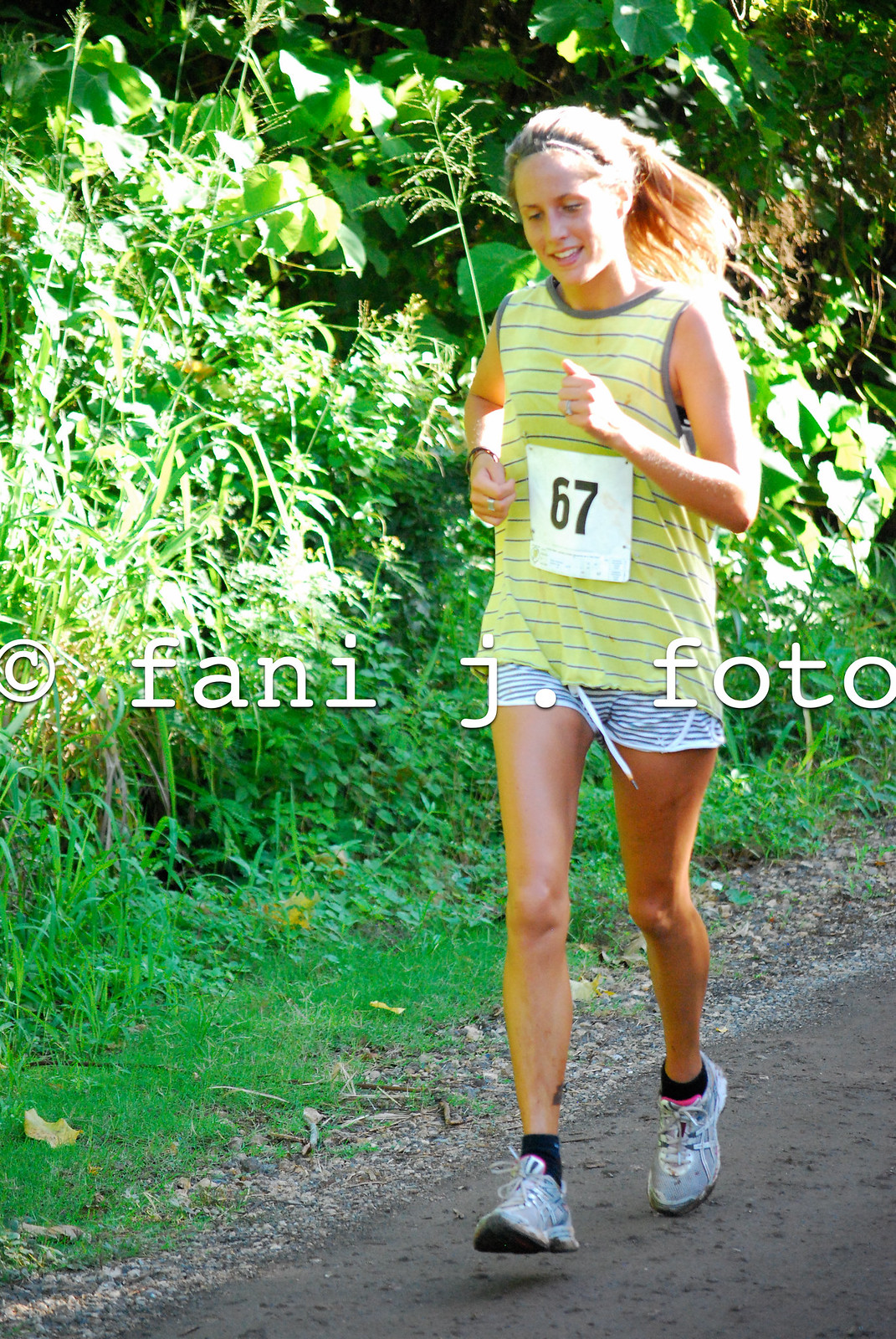In the image, a young woman, appearing to be between 15 to 20 years old, is captured jogging outdoors on a muddy or possibly rubberized trail. She is jogging towards the front-left of the frame with a slight smile on her face. Her blondish-brown hair, tied back in a ponytail, and a headband keeping it in place, moves slightly with her motion. She is wearing a sleeveless yellow tank top with gray horizontal stripes and a white square pinned to her chest displaying the number 67 in bold black letters, indicating she is participating in a race or marathon. Her shorts are blue and white striped, paired with black ankle socks and gray running shoes with blue and white accents. 

The background of the image is lush and green, with a mix of overgrown grasses, bushes, and tall leafy plants, suggesting a wooded or garden area. The path she runs on appears to be dark gray, possibly wet dirt or asphalt. The scene is lit by sunlight, adding brightness to the greenery. Across the middle of the image, there is a watermark that reads "Fanny J. Foto" in white, indicating the photographer. Her stride is captured mid-motion, emphasizing the dynamic nature of the activity.